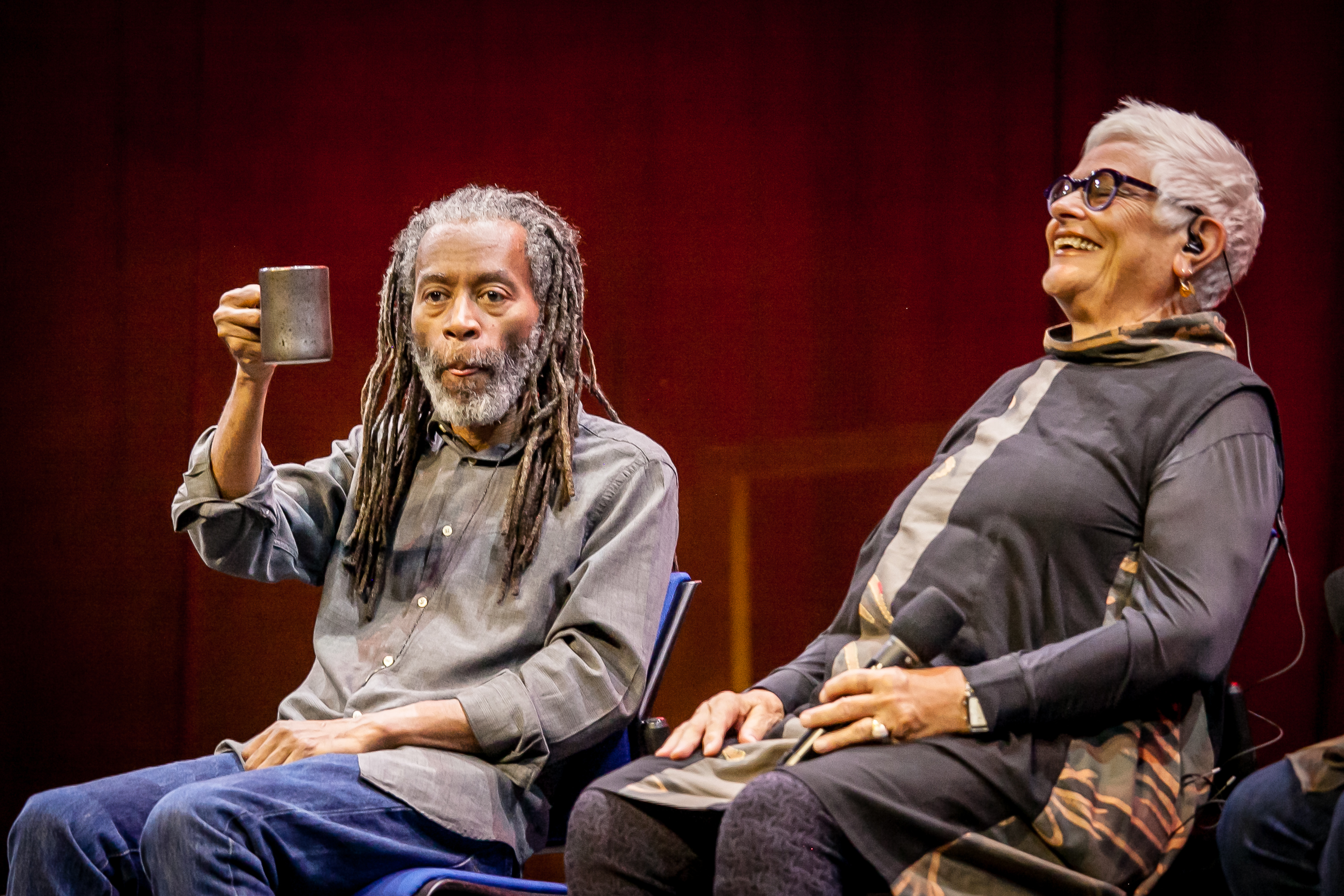In this image, Bobby McFerrin, a renowned musician, is seated on the left side. Bobby is a black man likely in his late 60s or early 70s, characterized by his gray beard, mustache, and long silver dreadlocks that fall across his chest. He is dressed in a grayish-green button-up shirt with long sleeves and blue jeans. Bobby holds a gray metal coffee mug in his right hand, seemingly in a gesture of 'cheers' to someone in the audience, while his left hand rests on his lap.

To Bobby’s right, an elderly woman is seated, leaning back and laughing heartily. She has short silver hair and wears thick black-framed glasses. Her attire includes a long dark tunic with a gray stripe and gray leggings, and she holds a microphone in her left hand, with an earpiece visible in her ear. Her right hand rests on her lap. The setting features a background with a cherry wood color, adding to the warm and engaging atmosphere of the scene. In the lower right corner, one can just glimpse the knees of another person.